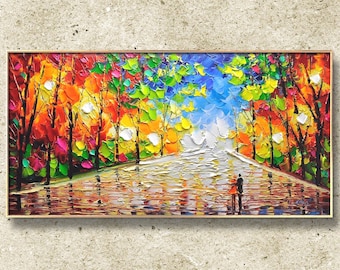This is a high-resolution photographic image of an oil painting displayed indoors on a marble or stone-like wall. The wall has a beige hue with white specks and some black dots, adding texture. The painting is enclosed in a thin wooden frame with a golden finish. The scene depicts a couple standing on a wide roadway, leading into the distance with a vanishing perspective. The woman, in an orange dress, and the man, in a black suit with his arm around her, have their backs to the viewer. They are positioned towards the lower center-right of the painting. The road is flanked by rows of trees on both sides, showcasing a vivid array of fall foliage with shades of orange, yellow, red, and some lingering green towards the center. The sky above is a clear, vibrant blue, and at the horizon, there are indistinct white blobs, possibly clouds or distant elements. The painting vividly captures the textures and brushstrokes, reflecting the artist's painterly style. There is no text present in the image.